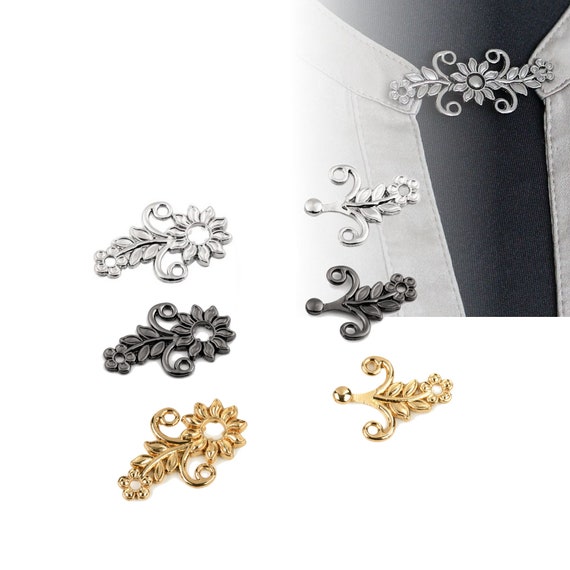The photograph displays seven decorative metal clasps designed to hold together the top of a jacket or blouse, particularly at the neckline, functioning almost like a choker. The clasps, which are shown on a white background, are made from various metals including silver, black, and gold tones, and are arranged in two columns with three rows of three different styles. Each row features the same design in different colors; the top row presents silver clasps, the middle row showcases black ones, and the bottom row displays gold-toned versions. On the left side of the image, three of these clasps are highlighted—one in silver, one in black, and one in gold. On the right side, a silver clasp is demonstrated on a black mannequin wearing a v-necked jacket or shirt, illustrating how the clasp, adorned with a flower design, fastens both sides of the collar together, creating a decorative focal point at the neckline.